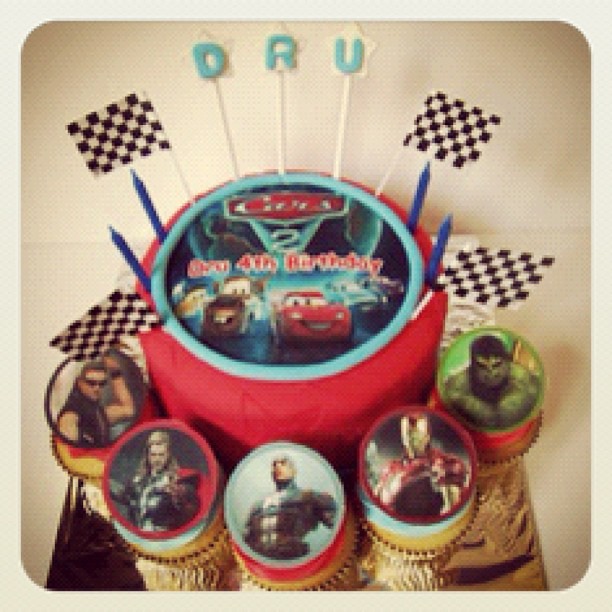This photograph depicts a vibrant birthday cake for Drew's fourth birthday, adorned with a Cars 2 theme. The main cake is a striking, saturated red and features a large, light blue circular topper that showcases cartoony cars from the movie "Cars 2," including red, brown, light blue, and dark blue vehicles. Around this centerpiece are four toothpicks with black and white checkered flags, possibly symbolizing a racing theme. Spelling out "DRU" are letters fixed on the top of the blue ring, each on a star-shaped background. The cake is accented with four navy blue candles, two on each side.

Surrounding the cake is a semicircle arrangement of cupcakes, each topped with printed images of Marvel superhero characters. Identifiable among them is the Hulk, while the rest remain indistinguishable. These cupcakes add to the festive theme, supported by what seems to be a reflective, square black dish beneath the cake. The backdrop of the image is a plain white, which might be a wall, table, or even a paper towel, emphasizing the vibrant colors of the cake and cupcakes against a neutral background. The overall impression is that of a lively and colorful celebration.